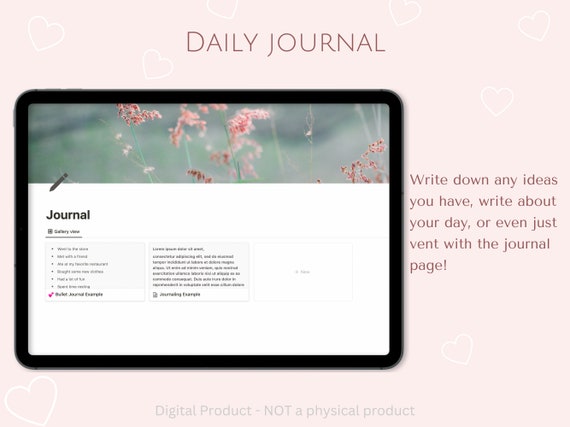The image showcases a visually appealing digital journal interface titled "Daily Journal" against a pink-themed background adorned with scattered white heart-shaped designs. At the top center of the image, bold text reads "Daily Journal," followed by a visual representation of a black-framed tablet. The tablet's display features an aesthetically pleasing cover image of blooming pink flowers set against a blurred green backdrop, reminiscent of grass. Below this floral cover, a section is designated for journaling, prominently marked with a pen icon and the word "Journal." Additionally, the journal template includes an example of a bullet journal, highlighted with two small heart icons. To the right of the digital journal, text guidance encourages users to write down ideas, document their day, or vent their feelings using the journal page. The footer of the image clearly states, in gray font, "Digital product, not a physical product," emphasizing its electronic nature.